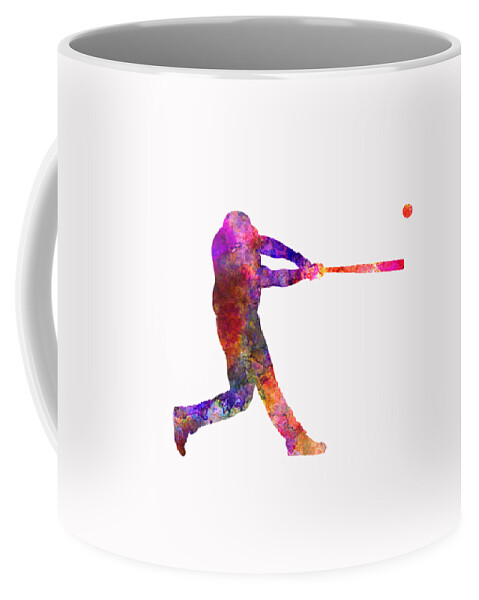This image features a basic white coffee cup with a light gray interior, depicted against a completely white background. The cup has a cylindrical shape with a visible handle on the left. The exterior of the cup showcases an abstract graphic of a baseball player. The player appears to have just hit a ball, with one leg bent and the bat extended in front of them. The bat, painted in vivid pink and orange hues, aligns with the ball, which is depicted as an orange dot above. The player’s silhouette is filled with a dynamic array of colors, including yellows, purples, oranges, blues, and browns, resembling a tie-dye or watercolor splash pattern. This colorful collage-like artwork contrasts with the simplicity of the white mug, making the design stand out prominently. Other than the cup with the vibrant baseball player design, the image contains no additional elements.